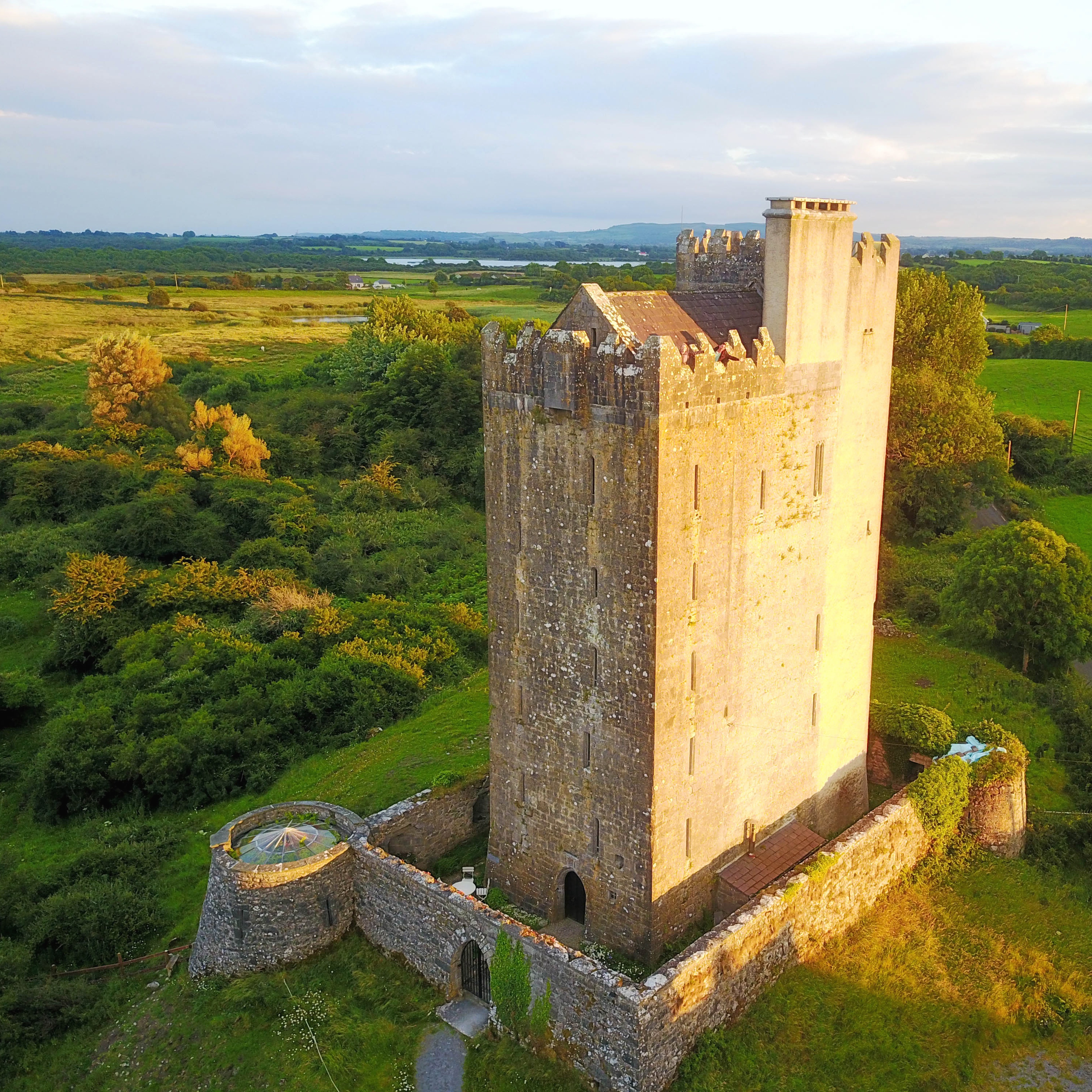The photograph captures a vertically rectangular image of a very old, tall stone building, reminiscent of a medieval castle, situated on a hill in the middle of nowhere. The imposing structure, constructed from golden-hued stones, stands out as a towering fortification surrounded by lush green fields, trees, and distant mountains, with a serene lake visible. This building, approximately six stories tall and notably thin, features vertical slits for windows and various decorations on the roof, including chimneys and a small turret. Enclosed by a one-story high stone wall adorned with green vines or moss, the fortress has two prominent outposts at the corners. A single doorway through the wall leads to a further entrance into the building, emphasizing its ancient and rudimentary design but conveying an impressive and steadfast presence in the tranquil countryside.